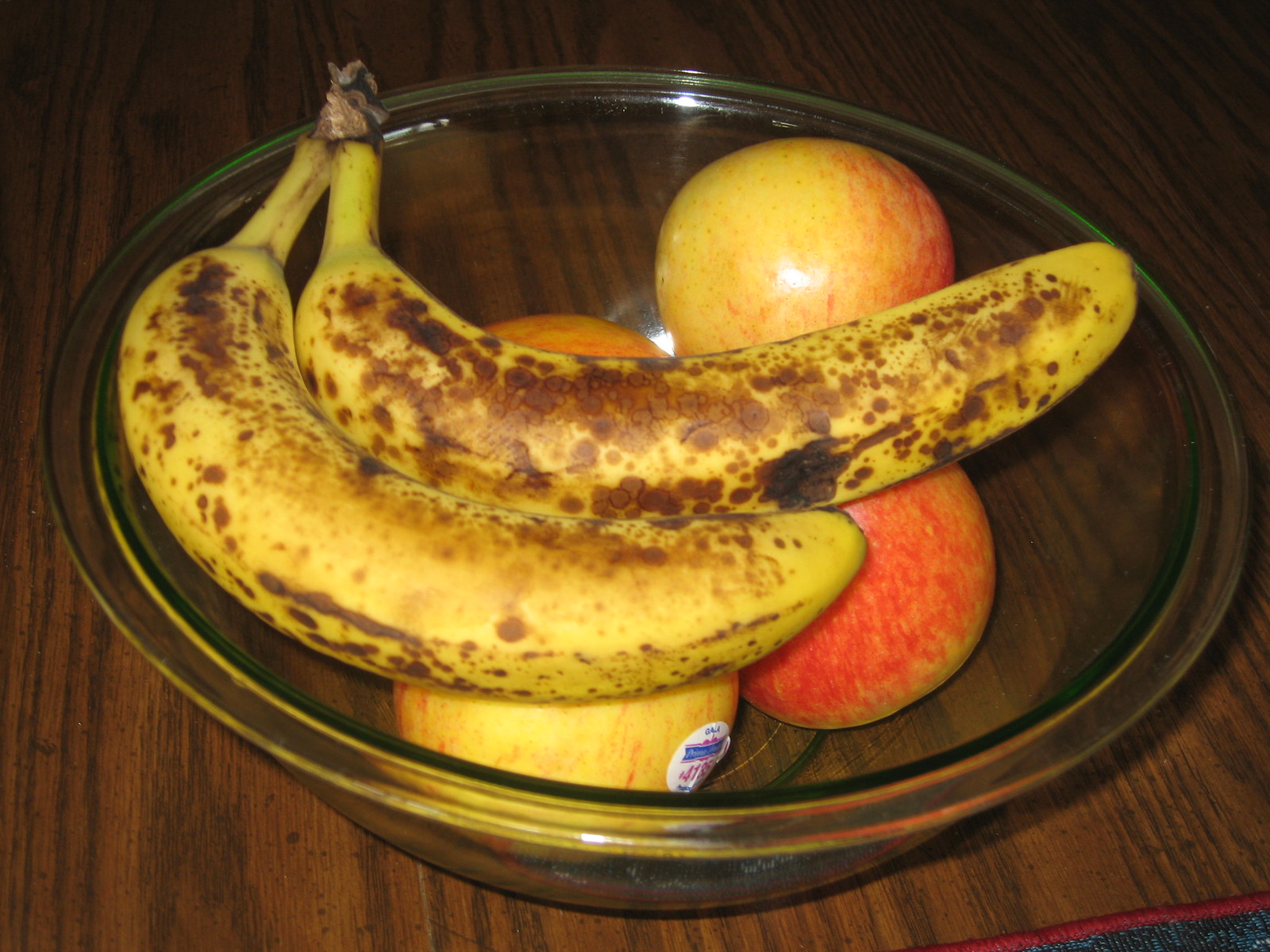A clear glass bowl filled with assorted fruits is prominently displayed on a dark wooden table. Inside the bowl, four apples are visible, each exhibiting a mix of red and yellow hues. One apple carries a fruit sticker, though it is too distant and indistinct to decipher the text. Atop the apples lie two yellow bananas, speckled with numerous brown spots, nearly covering their entire surfaces. In the bottom right corner of the frame, a small section of a placemat peeks into view. The placemat has a carpet-like texture, featuring a red-trimmed edge and a main body that appears to be a very dark green, blue, or black, though its exact color is challenging to determine.